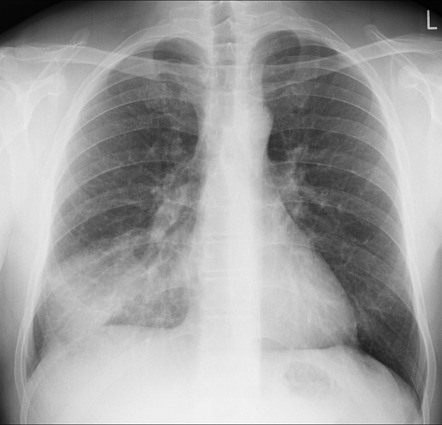This black and white image is a detailed chest x-ray of a person, capturing the anatomical structures from the shoulders down to the hips. Predominantly white against a black background, it clearly shows the rib cage, including the clavicle, the scapula bone, the central sternum, and the individual ribs. The spine is also visible, along with parts of the neck bone and the shoulder bones. The image depicts several internal organs, such as the heart, the lungs, and the diaphragm, which may also suggest the diaphragm or the liver. A distinctive white 'L' can be seen prominently in the top right-hand corner of the x-ray. This image is typically used in a medical context, likely for patient diagnosis in a hospital setting. The empty spaces between the ribs and around the body are dark, providing contrast to the skeletal details.